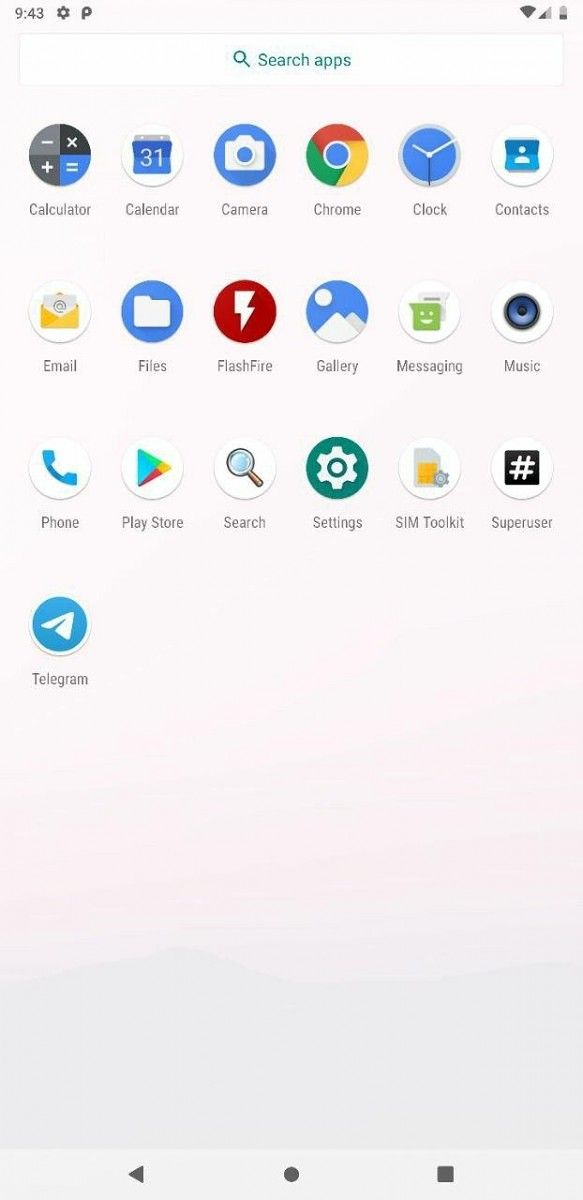Screenshot of a smartphone home screen displaying the time as 9:43 AM. Various app icons are visible, including Google, Calculator, Calendar, Camera, Chrome, Clock, Contacts, Email, Files, Flash Fire, Gallery, Messaging, Music, Phone, Play Store, Search, Settings, Smart Toolkit, Super User, and Telegram. The background is gray, adorned with a black square, black circle, and black triangle. The top right corner shows status icons including a black Wi-Fi symbol, a black cell phone service symbol, and a nearly depleted black battery symbol estimated to be around 28-34%. A settings wheel is located at the top alongside the time. Additionally, there appears to be a black icon with characters resembling "P" and "Jingzong Zee Jingao" next to the time.